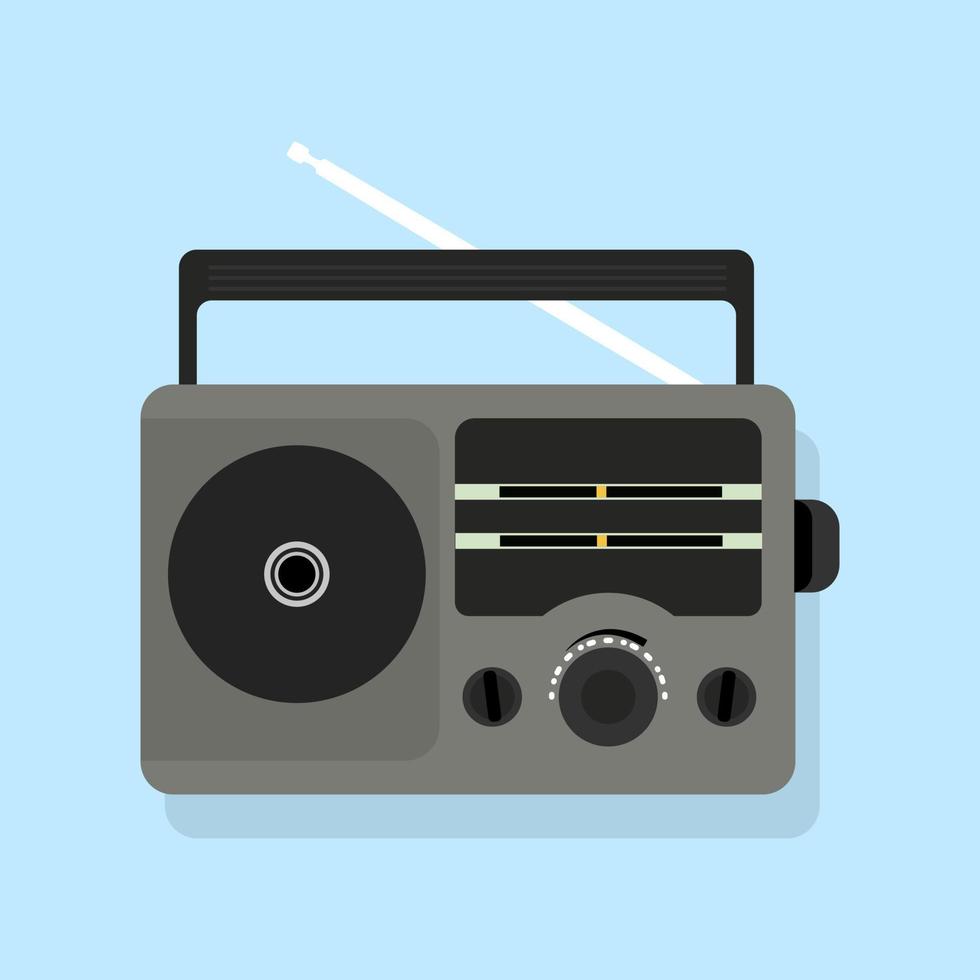The image is a computer-generated, stylized poster featuring an old-fashioned portable transistor radio, rendered against a baby blue background. The radio, centrally placed with a shadow cast in a darker shade of blue, is primarily gray with various darker gray tones accentuating its features. A black handle on top and a white antenna extending diagonally upwards are clearly visible. The radio showcases a large black speaker and several operational knobs: three main dials, including one with white dashes for tuning intensity, and additional black and gray knobs likely for volume and station tuning. Two small horizontal bars adjacent to the tuning knob suggest dual functionality, possibly for switching between AM and FM frequencies. Intricately drawn, the detailed depiction emphasizes the contrast between the black and gray components, enhancing the vintage appeal of the radio.